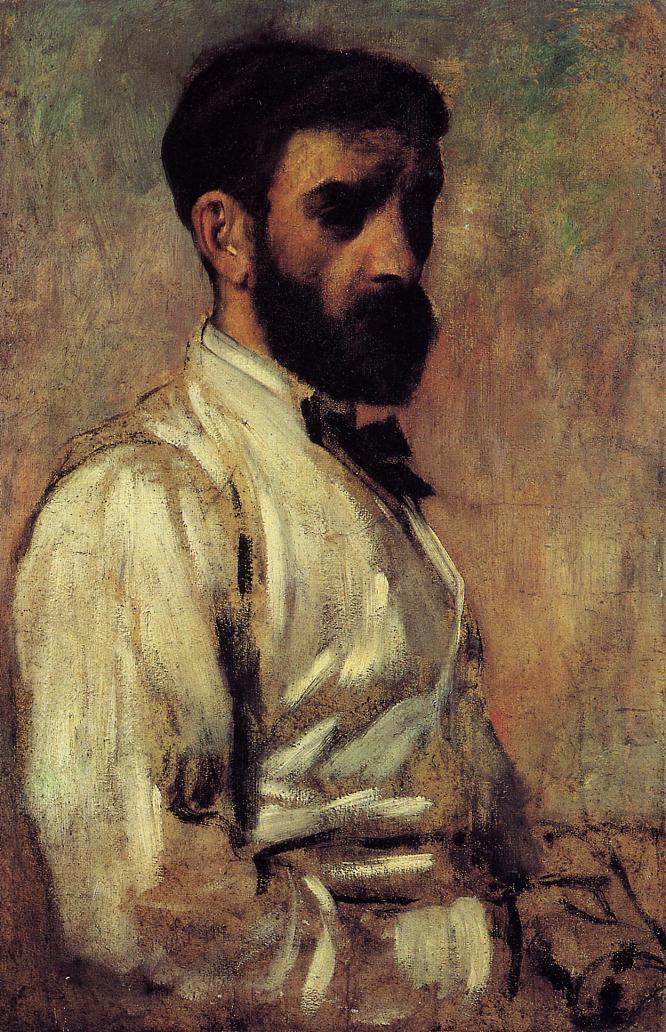The image depicts a painting, likely a portrait, of a man positioned centrally and occupying most of the frame. The background is a multicolored blend that contrasts with the figure. The man, seated and shown from the waist up, is in a side profile facing the right, yet looking towards the painter. He has thick, dark hair combed to one side and a well-trimmed, bushy beard. His face, characterized by somewhat sunken cheeks, is largely in shadow, obscuring his eyes and lips. He is dressed in a clean, white long-sleeve shirt paired with a dark bow tie, exuding an early 20th-century elegance. The shadows and lighting suggest an olive-skinned complexion, though this could also be due to the painting's stylistic choices. His pose is relaxed, with at least one hand casually placed in his pocket, adding a touch of informality to the otherwise formal attire. This art piece appears suited to a museum or an art show setting.